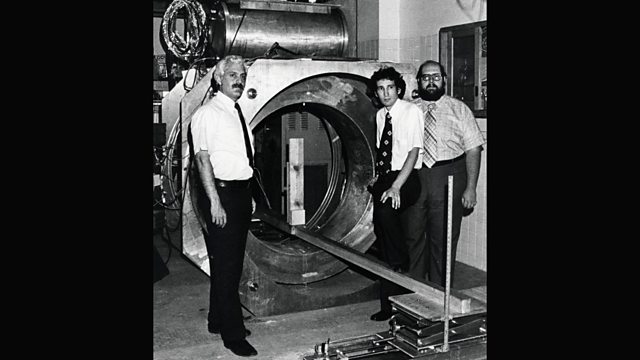The image features a black and white photograph with black borders on the left and right, creating a letterbox effect. Central to the photograph is a bulky, tube-like device, approximately four feet in diameter, facing the viewer. This large metal contraption appears to be an old type of MRI machine, characterized by its circular structure and a thin metal rail visible inside.

Three men are positioned in front of the machine. On the left stands an older man with white, short, curly hair and a dark mustache. He is dressed in a white, short-sleeved button-up shirt, a black tie, black pants, and black shoes. To his right are two younger men. The first wears a white shirt with a polka dot tie, black pants, and black shoes, and has curly black hair. The second, standing on the far right, is slightly overweight, has a full beard and mustache, is balding at the front with black hair at the back, and wears glasses. He is dressed in a pinstripe shirt, a checkered black and white tie, gray pants, and a black belt. The overall scene captures a moment of interaction among the men and this intriguing piece of historical medical equipment.